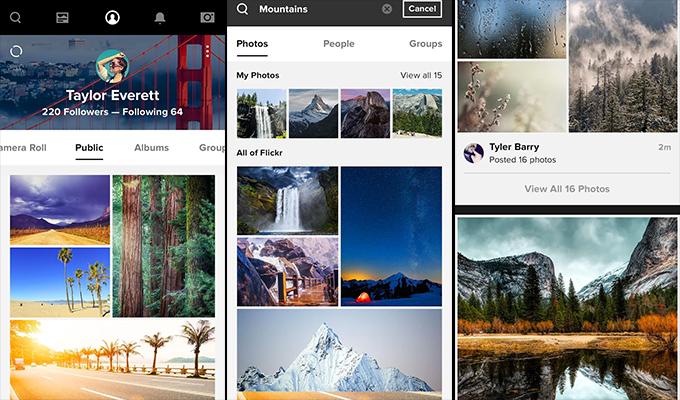On Taylor Everett's social media profile, she boasts 220 followers and follows 64 people. Her profile is represented by a small turquoise thumbnail showing her picture. The latest post features a variety of photos from her holidays, curated into several themed sections. The main section is titled "Mountains," featuring breathtaking landscapes including a striking red superstructure that seems to carry power lines, several majestic mountain ranges, a serene night sky over mountains, and multiple cascading waterfalls, one of which flows down towards a quaint bridge nestled in the mountains.

Scrolling down further, a variety of other picturesque captures appear under the heading 'Photos.' These include captivating images of tropical locations with lush palm trees, a dense pine forest, and a striking snow-covered mountain, reminiscent of the Himalayas due to its sharp, pointed peak. Additionally, there's a collection labeled 'All of Flickr,' showcasing a diverse mix of nature's beauty. Also noteworthy is a series of 16 photographs posted by another user named Tyler Barry, complementing Taylor's extensive album.